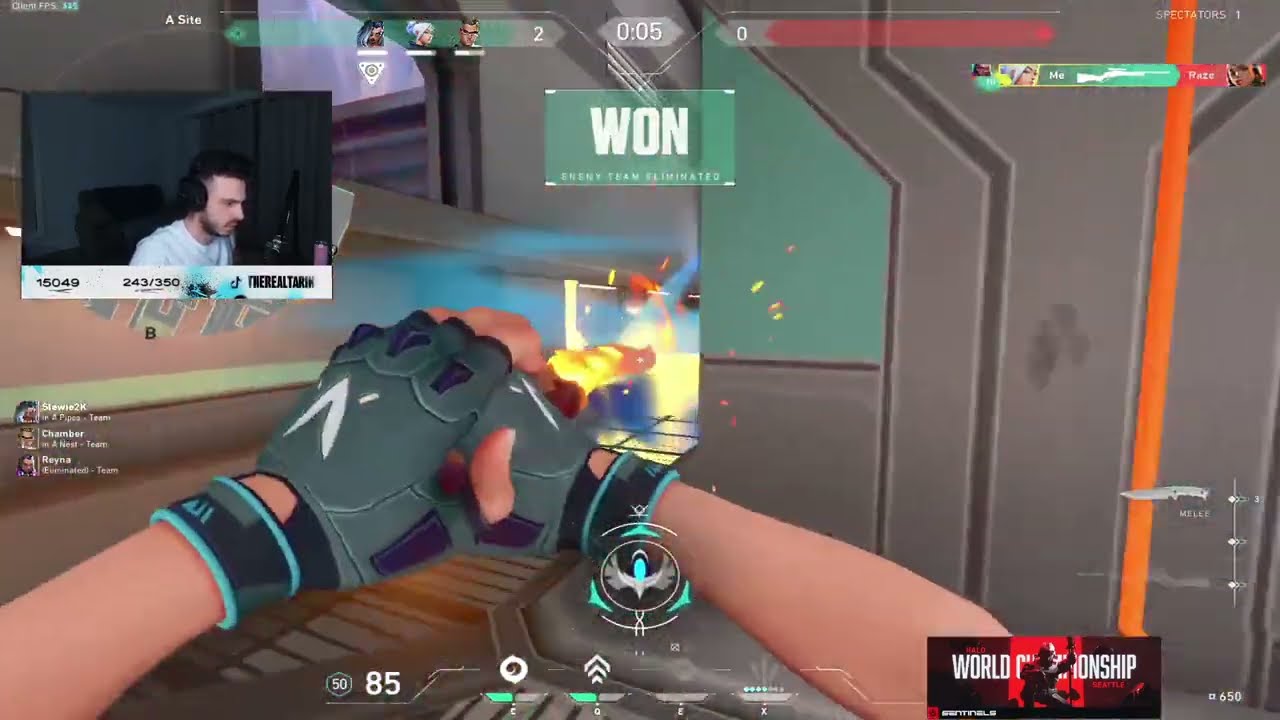The image depicts a first-person shooter video game screenshot being live-streamed by a player. At the center of the image, the player's gloved hands, wearing gray fingerless biker gloves, are extended outward, emitting fire down a metallic spaceship-like hallway. The hallway features metal panels on the doors, with a metal walkway on the left and cargo bay doors to the right. The setting is industrial, evoking a high-tech, futuristic ambience.

In the top left corner, a picture-in-picture frame shows the live-streamer, a white man with black hair, wearing a white t-shirt and headphones. He is intensely focused on his screen in a dark room with a brown-black wall behind him. 

The image includes various texts, with "1" in a green box in the middle of the screen, and "Enemy team eliminated" along with "World Championship" in a red and black banner at the bottom. The color palette of the scene includes black, white, gray, light blue, green, orange, red, and yellow, adding to the dynamic and immersive visual experience.